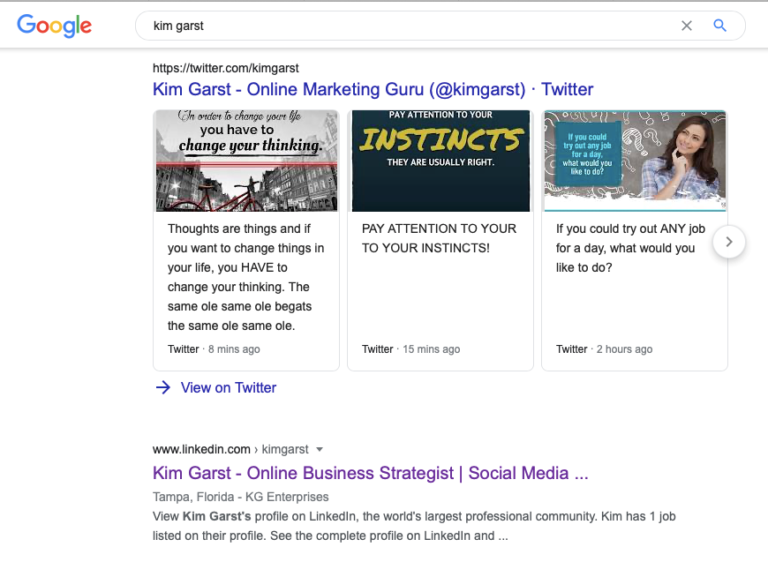The provided image is a screenshot taken on a laptop or desktop computer, showcasing a Google search results page. The visible portion of the screen excludes the browser interface, making it difficult to determine the specific browser in use. Central to the image is the Google homepage, featuring the iconic multicolored Google logo at the top left. To the right of the logo is a search bar displaying the query "Kim Garst," with a magnifying glass (search) button and an 'X' (clear) button adjacent to it.

The search results for "Kim Garst" are prominently displayed. The top result links to Kim Garst's Twitter account, including highlighted tweets such as:
- "Thoughts are things, and if you want to change things in your life, you have to change your thinking."
- "The same old, same old, begets the same old, same old."
- "Pay attention to your instincts."
- "If you could try any job for a day, what would you like to do?"

Beneath the Twitter link, the second result is for Kim Garst's LinkedIn profile. The descriptive snippet underlines her professional exposure, stating: "Kim Garst, online business strategist, social media, Tampa, Florida, KG Enterprises. View Kim Garst's profile on LinkedIn, the world's largest professional community. Kim has one job listed on their profile. See the complete profile on LinkedIn."

The webpage's background is a clean white, with black text alongside blue hyperlinks, ensuring readability and a professional look. The image is captured in a standard 4:3 aspect ratio, providing a comprehensive view of the search results and their layout.